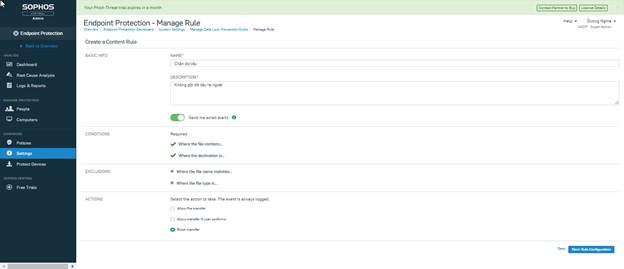The image depicts a web page that appears to be an administrative dashboard for a software application. The interface features a black vertical menu on the left side with white text, displaying options such as "SOPHOS," "Dashboard," "People," and "Computers." The central part of the page includes a top section with two unidentified buttons on the right-hand side and some introductory text against a light green background on the left. Below this, there is a heading labeled "Endpoint Protection Manage Rule," with some accompanying descriptive text to its right. Further down, the page shows a form section titled "Create a Content Rule" with subsections like "Basic Info," containing text input fields. The text in various parts of the image is either too small or too blurry to be clearly identified.